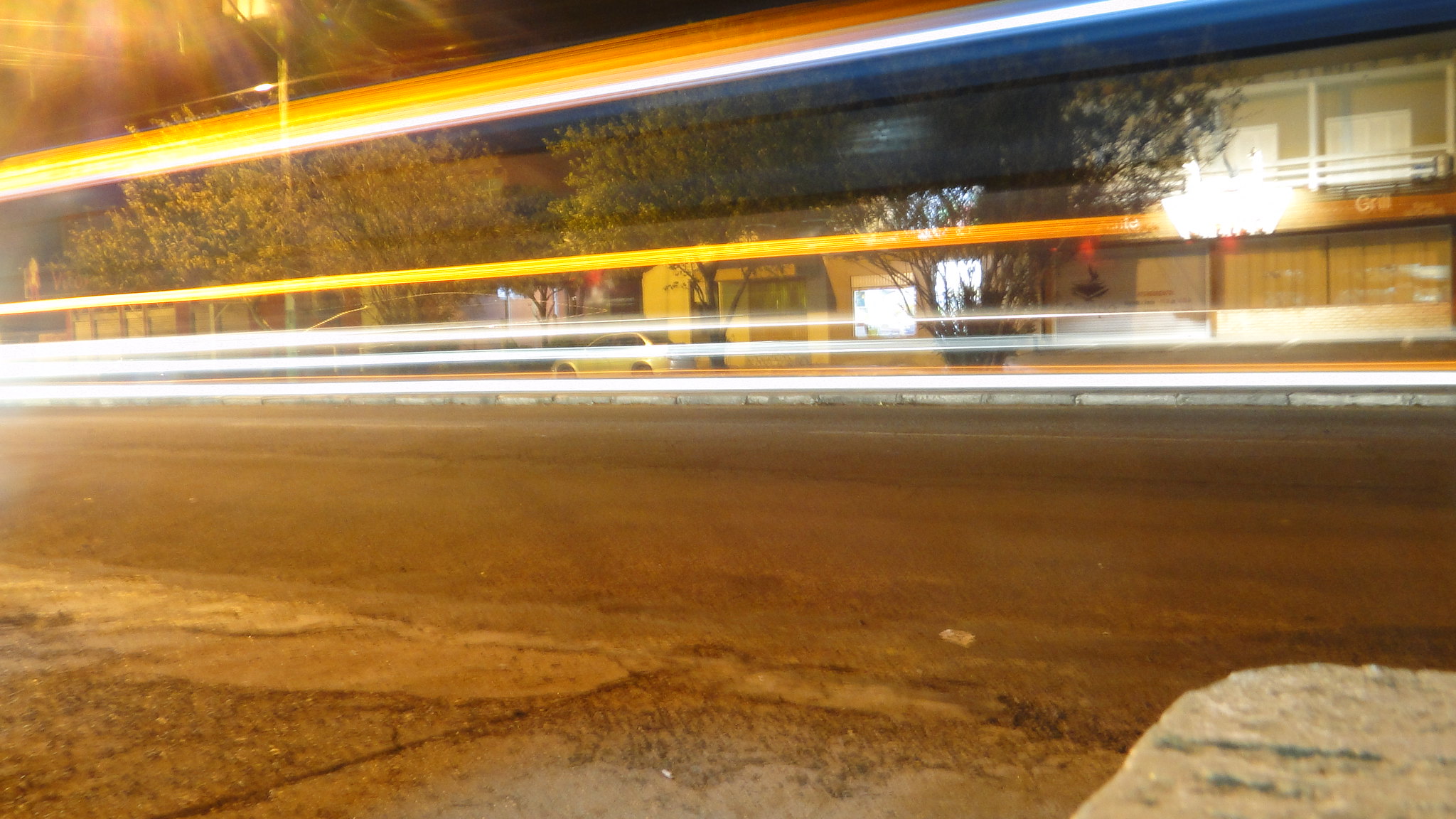This detailed nighttime or early morning photograph captures a city street scene, highlighting the dynamic yet serene nature of urban life. The gray asphalt street, slightly worn and cracked, extends from the bottom of the image, bordered by what appear to be small businesses or apartment buildings in white or tan hues towards the top. A parked car sits in front of these buildings, partially obscured by several trees with brown trunks and green leaves. 

On the left side, a tall street light emits a warm yellow glow, illuminating the surroundings faintly against the dark sky. The standout feature of the photograph is its long-exposure effect, capturing the motion of a speeding car through the brilliant trailing lights. These streaks, comprising two yellowish-orange lines above and three white lines below, span horizontally across the frame from left to right, vividly depicting the car's rapid passage.

In the distance, the buildings' structure is more apparent, showcasing white trims and windows with five or six bushes lined up in front. The lower right corner subtly shows a curb or possibly a rock, adding to the street's textured detail. The entire scene, illuminated softly yet dynamically, evokes the bustling yet still moments of an urban night.